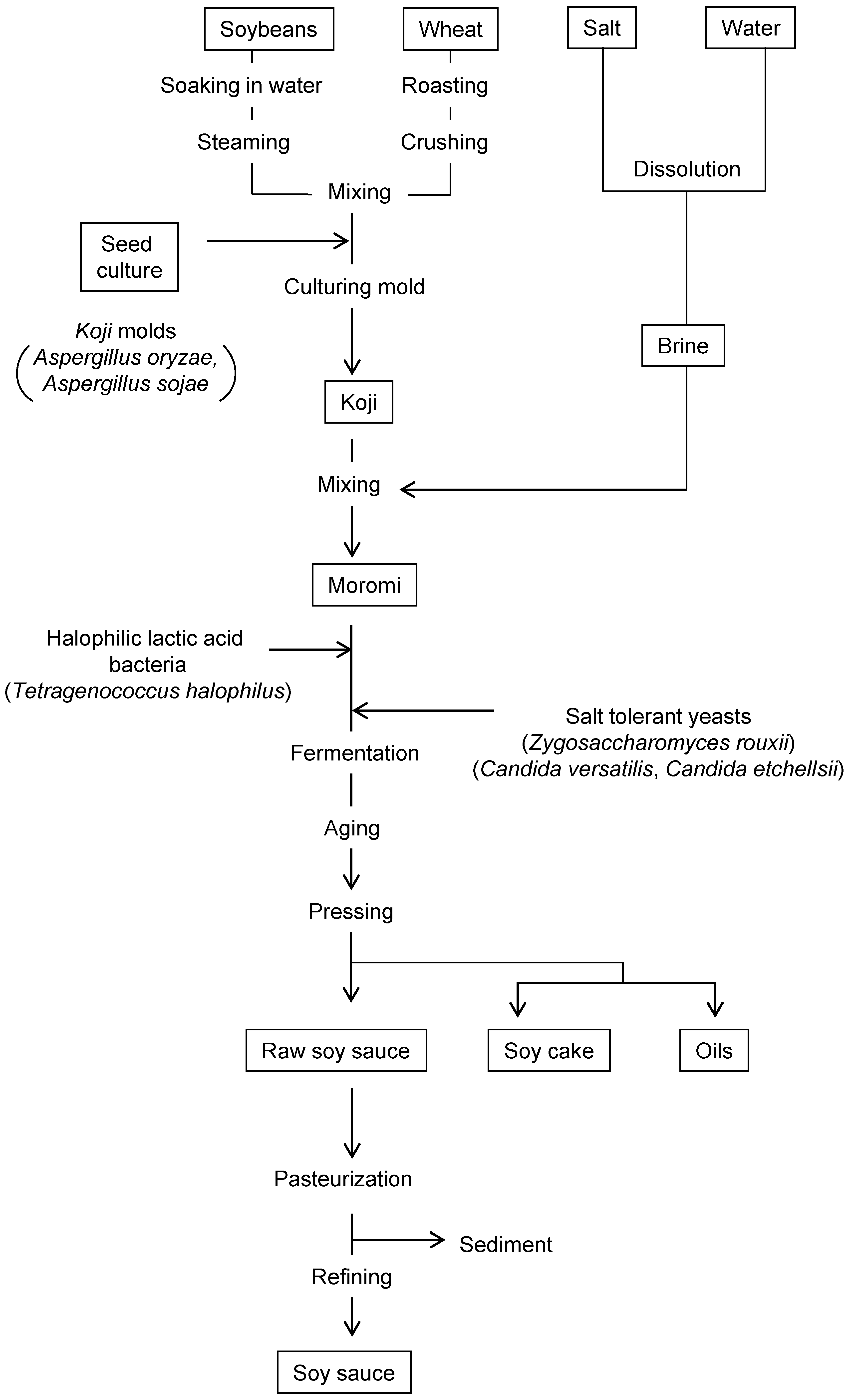This detailed flowchart on a white background with black lettering and outlines illustrates the comprehensive process of transforming soybeans, wheat, salt, and water into soy sauce. The diagram initiates with four main labels at the top: soybeans, wheat, salt, and water. Moving downward, the soybeans undergo soaking in water, steaming, and are then combined with wheat that has been roasted and crushed. These processes culminate in a mixing stage.

Adjacent to this, salt and water merge at a later stage to form a brine through dissolution. This brine then integrates with the mixed soybeans and wheat at the koji stage, where a culturing mold is introduced. The mixture proceeds through several sequential steps: creating moromi, followed by fermentation, aging, and pressing.

Post-pressing, the flowchart diverges briefly, indicating that one path leads to either soy cake or oils, while the main path continues towards raw soy sauce. Finally, the raw soy sauce undergoes pasteurization and refining before reaching the end point, labeled simply as soy sauce. The chart meticulously tracks each transformation and interaction of the initial elements, culminating in the production of soy sauce.